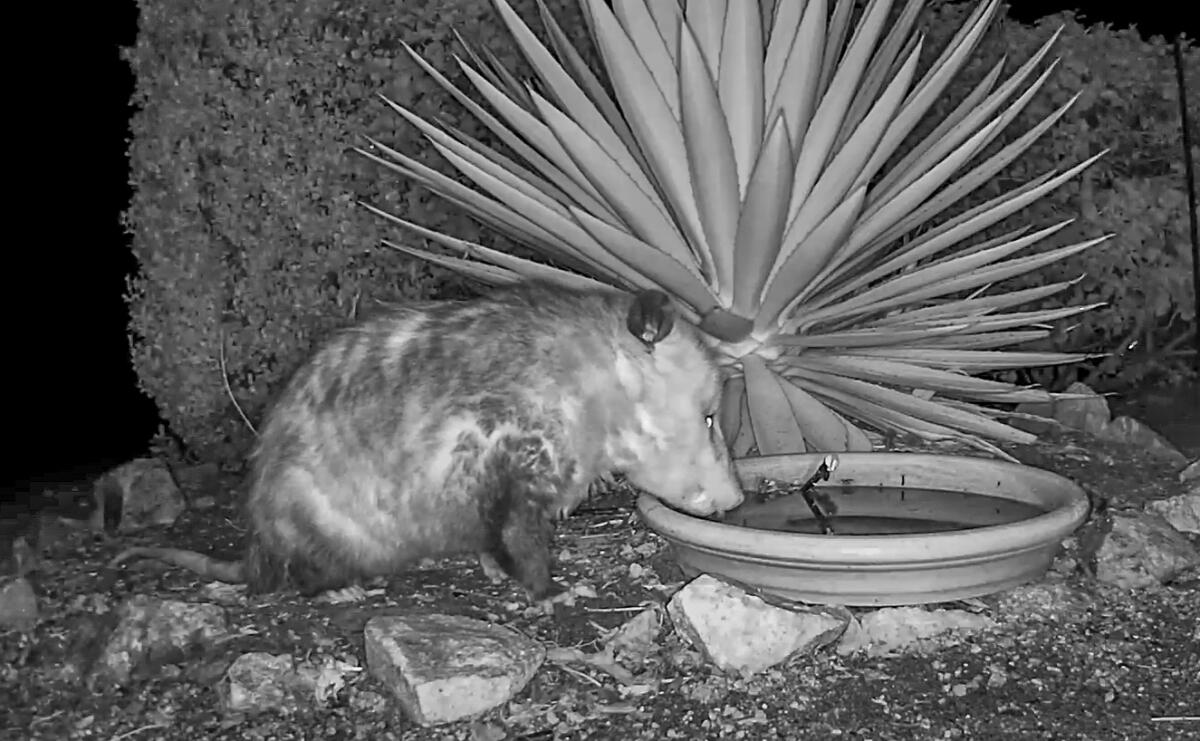In this black and white photograph, likely captured by a night vision security or ring camera, a possum is seen drinking water from a shallow bowl placed on the ground. The possum's eyes reflect the camera's flash, creating a glowing effect. The scene is set in what appears to be a garden area, with dirt and small rocks scattered around. In the background, there are shrubs and a plant with spike-like leaves, possibly an agave or cactus. The possum, identified by its distinctive face and tail, seems intent on hydrating itself from the bowl, which might have been initially placed for another animal, such as a dog. This surprise visitor adds a touch of wildlife charm to the garden setting at night.